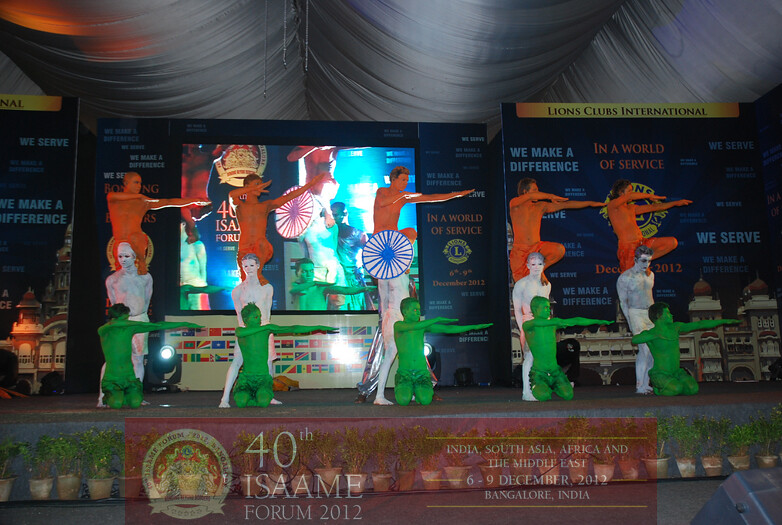The image features a stage setup with fifteen performers arranged in a visually striking formation. The backdrop is filled with various advertisement displays featuring blue panels inscribed with numerous words. Hanging above the scene are silver-gray curtains, drooping to form three semi-circular shapes. The stage itself is slightly elevated with a light gray floor, adorned in front with small green plants in red pots. The performers, all male, are painted head-to-toe in three distinct colors: green, white, and red (or orange). The performers are divided into three rows, each row consisting of five individuals. The front row, painted green, kneels on the stage with their arms extended to the left. The middle row, painted white, stands behind them in a semi-kneeling position with their arms resting straight down. The back row, painted red (or orange), stands at a higher elevation with one leg bent and their arms also extending to the left. At the bottom of the image, text overlays mention the "40th ISAAME Forum 2012," detailing the event’s location and dates: "India, South Asia, Africa, and the Middle East, 6 to 9 December 2012, Bangalore, India."